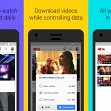This image appears to be a small, possibly low-resolution advertisement for a mobile application. The layout is divided into three vertical sections, each featuring a different background color and a smartphone image. 

On the left, a purple background emphasizes a smartphone displaying an app screen. The center section, with a yellow background, showcases another smartphone highlighted by a pop-up notification within the app. The central text is somewhat legible and suggests, "Download video while controlling data." The right section has a light blue background and another smartphone image, but the text here is cut off and unreadable. 

The colors in the advertisement include shades of bluish-purple, light blue, yellow, black, and white. This ad aims to promote a mobile app, likely related to managing downloads and controlling data usage. Writing at the top of the image is too small to decipher, and further details in the pop-up notification are not clear due to the tiny size of the image.